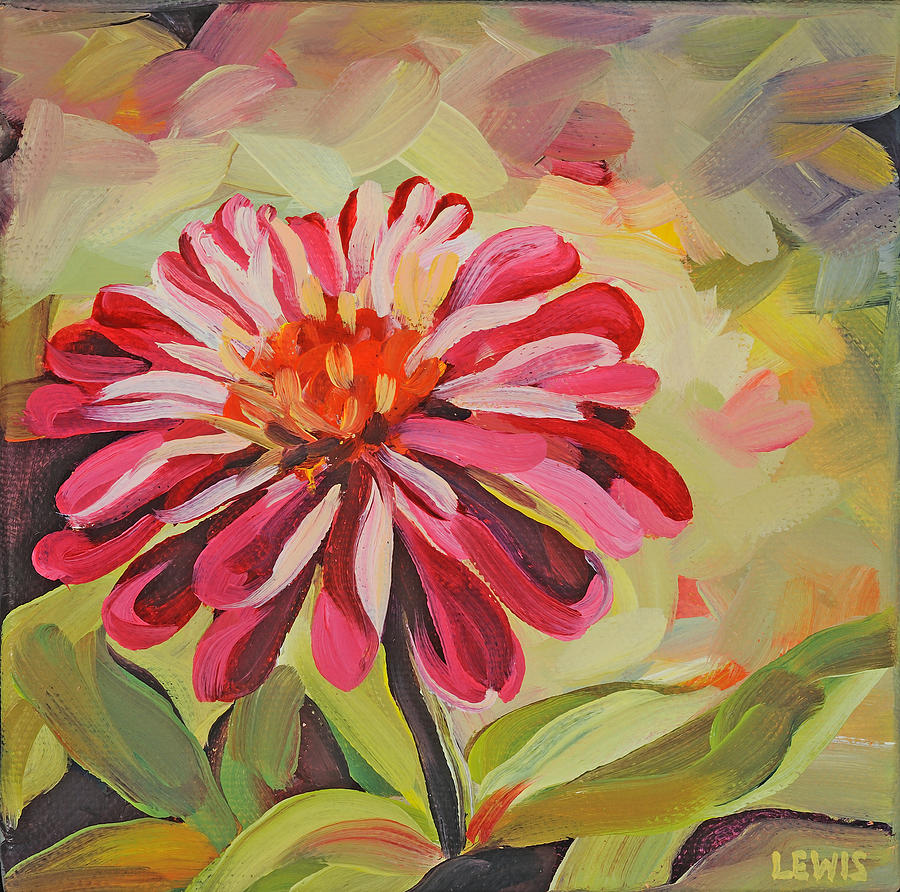This artwork is a detailed and vibrant painting of a flower, prominently featuring a bold and striking bloom with red, pink, and white petals and a bright orange-yellow center. The flower stands out in the foreground, positioned slightly to the left, and immediately draws the viewer's gaze. The stem is painted in a dark green, and it is surrounded by a mix of richly colored leaves and a backdrop of diverse hues, including pastel purples, pinks, creams, and yellows. This blend of colors gives the background a soft, romantic feel, enhancing the overall visual appeal. The name "Louis" is elegantly signed in yellow in the bottom right-hand corner, likely indicating the artist. This slightly abstract watercolor painting exudes a sense of softness and beauty in its harmonious use of color and form.